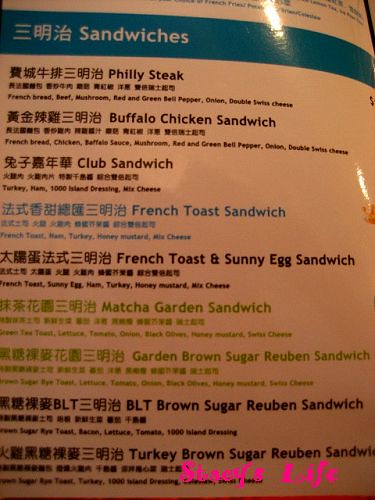The image depicts a restaurant menu, likely from an Asian (possibly Chinese) establishment, as indicated by the presence of Chinese characters on the left side of the menu, with English translations on the right. The menu is topped with a blue banner featuring the sandwich offerings in white font. A detailed description of the sandwiches follows:

1. **Philly Cheesesteak:** French bread, beef, mushrooms, red and green bell peppers, onions, and double Swiss cheese.
2. **Buffalo Chicken Sandwich:** French bread, chicken, buffalo sauce, mushrooms, red and green bell peppers, onions, and double Swiss cheese.
3. **Club Sandwich:** Turkey, ham, Thousand Island dressing, and mixed cheese.
4. **French Toast Sandwich:** French toast, ham, turkey, honey mustard, and mixed cheese (highlighted in blue font).
5. **French Toast and Sunny Egg Sandwich:** French toast, sunny-side-up egg, ham, turkey, honey mustard, and mixed cheese.
6. **Matcha Garden Sandwich:** Green tea toast, lettuce, tomato, onion, black olives, honey mustard, and Swiss cheese (highlighted in green font).
7. **Garden Brown Sugar Reuben Sandwich:** Details are blurry, making it difficult to read.

Additionally, the menu lists:
8. **BLT Brown Sugar Reuben Sandwich**
9. **Turkey Brown Sugar Reuben Sandwich**

The image appears to originate from a source associated with "Stacy's Life."